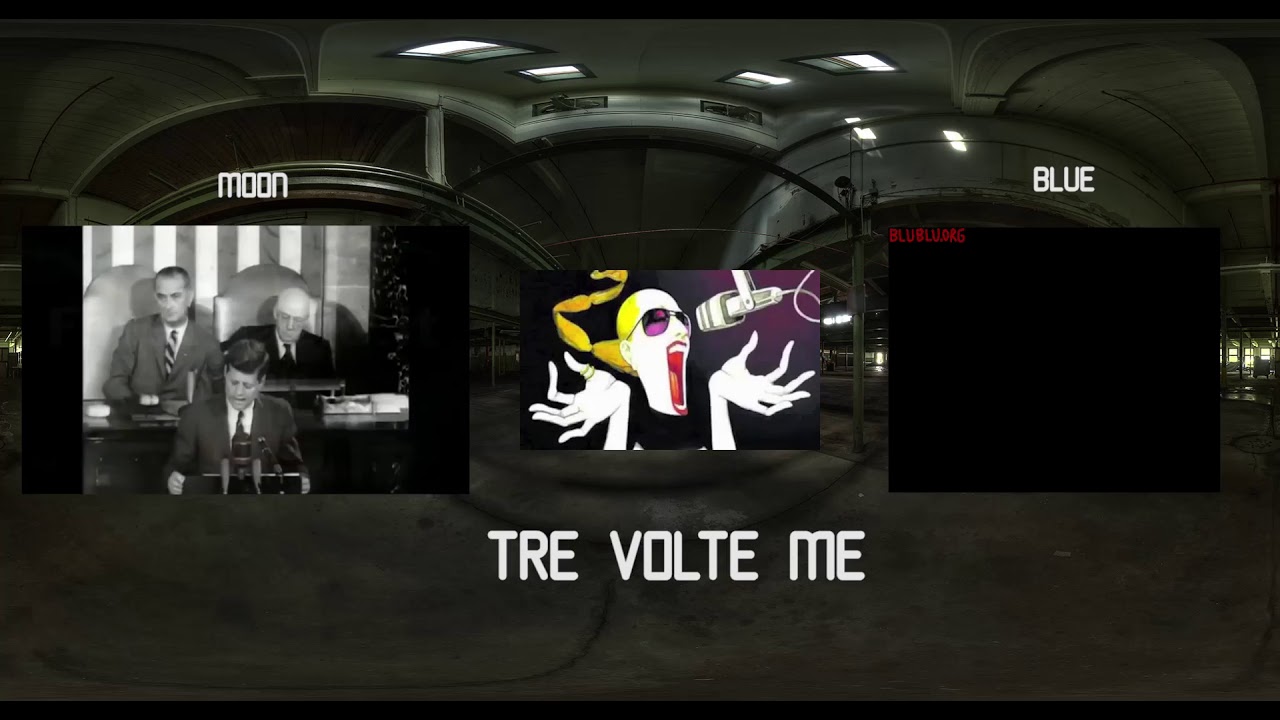This collage-style image features a composite background that appears to be a wide-angle, somewhat distorted photograph of an urban subway or cityscape. On the left side, there is a black-and-white photograph labeled "moon" at the top. The photo prominently features John F. Kennedy delivering his famous Moon landing speech, with Vice President Lyndon B. Johnson seated behind him and another unidentified government official. 

In the center of the image, there's a detailed cartoon of a rock singer with a white face, yellow ponytail, and purple glasses, animatedly screaming into a microphone. Accompanying this drawing are the artist's hands, which are outstretched, further enhancing the sense of dynamic performance. Below this drawing, in large, bold white text, is the caption "T-R-E-B-O-L-T-E me."

On the right side, there's a stark black rectangle labeled "blue" at the top, with some red letters in the top-left corner reading "blue vorg" or possibly "blue blue org," although this section is somewhat ambiguous due to the abstract nature of the image. This overall artistic composition balances historical photography with modern, expressive illustration, set against a mysterious urban backdrop.